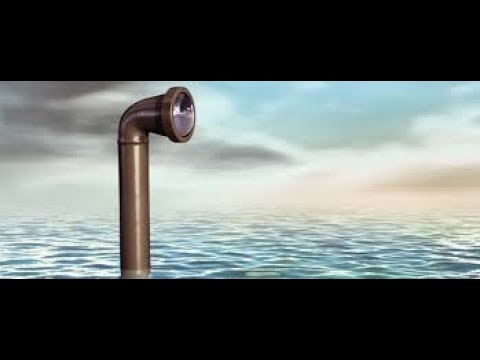The image features a visually striking scene, reminiscent of a cinematic frame with black widescreen bars stretching across the top and bottom. At the center of this aquatic setting, a bronze-colored periscope emerges from the tranquil water, designed with a shiny brownish metal and a forward-facing lens reflecting the clear blue sky. Positioned on the left side of the photo and angled to the right, the periscope captures a detailed view, suggesting an animated movie-like rendering. The water below spans a spectrum of light blue, turquoise, and green hues marked by gentle, almost imperceptible waves. This serene expanse meets a horizon where the sky reveals a contrast: on the left, dark gray, rain-laden clouds hint at a potential storm, while on the right, the sky opens up to a peaceful scene of light blue with fluffy white clouds interspersed with an orange glow, evoking a picturesque transition, perhaps of dawn or dusk.